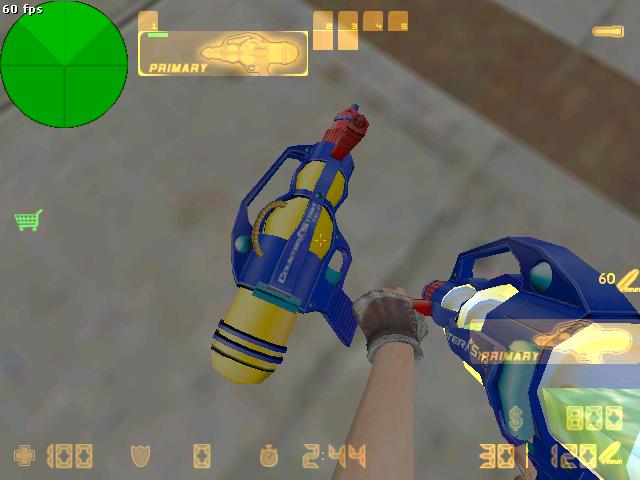In the image, we see a screenshot from a video game, although the specific game is not identified. The top left corner displays white text reading "60 FPS," indicating the game runs at 60 frames per second. Below this text is a green circular map or compass, which is divided into four quadrants, but no specific details are visible on it. Directly beneath the compass, there is a green icon of a shopping cart.

Moving to the very bottom left corner, there is a yellowish-brown health symbol depicted as a cross, accompanied by the number "100," indicating the player has full health. Adjacent to this, a shield icon representing armor shows a value of "0," meaning the player has no armor. Additionally, a stopwatch icon is visible in this corner.

At the bottom center of the screen, a clock stopwatch icon shows "2:44," likely referring to the elapsed or remaining time in the game. Over on the bottom right, a money symbol is displayed with a value of "$800." Below this, ammunition details are provided: "30" rounds are currently equipped, while "120" rounds are available for use. These numbers are separated by a line.

In terms of in-game context, the player appears to be holding a weapon, which resembles a water gun, in one hand, while a similar weapon lies on the ground. The player's hand, covered by a brown glove, is visible at the bottom of the screen, indicating they are looking down at the weapon on the ground.